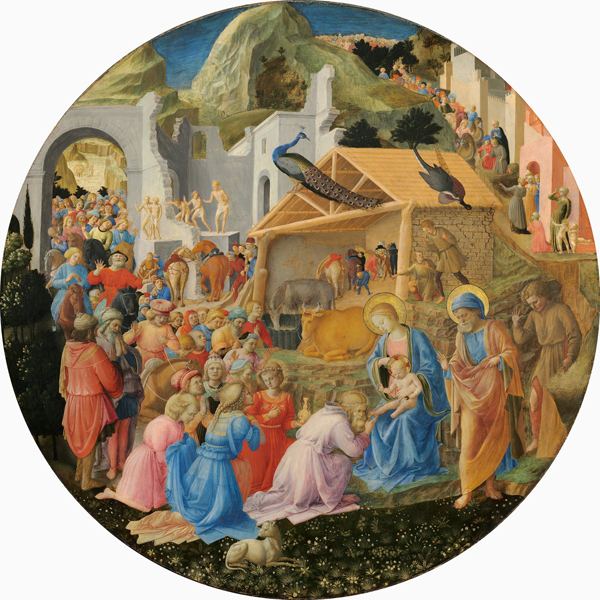The painting is a highly detailed, circular oil artwork reminiscent of Renaissance design depicting the nativity scene. At the center-left, a woman in a blue robe, likely Mary, holds a baby, presumably Jesus, both adorned with golden halos. Beside her stands an elderly man, dressed in a pinkish-coral robe and a blue headdress, also with a halo, signifying Joseph. The scene is bustling with about a hundred people, many kneeling in reverence before the holy family. The background features a stable with various animals, including a cow, a deer, and a distant, distinct peacock perched on the barn. A gateway can be seen in the distance, from which more people are arriving, some on a ramp that suggests a one-way passage. The detailed depiction of vibrant, colorful figures enriches the spiritual and celebratory atmosphere of the birth of Christ.